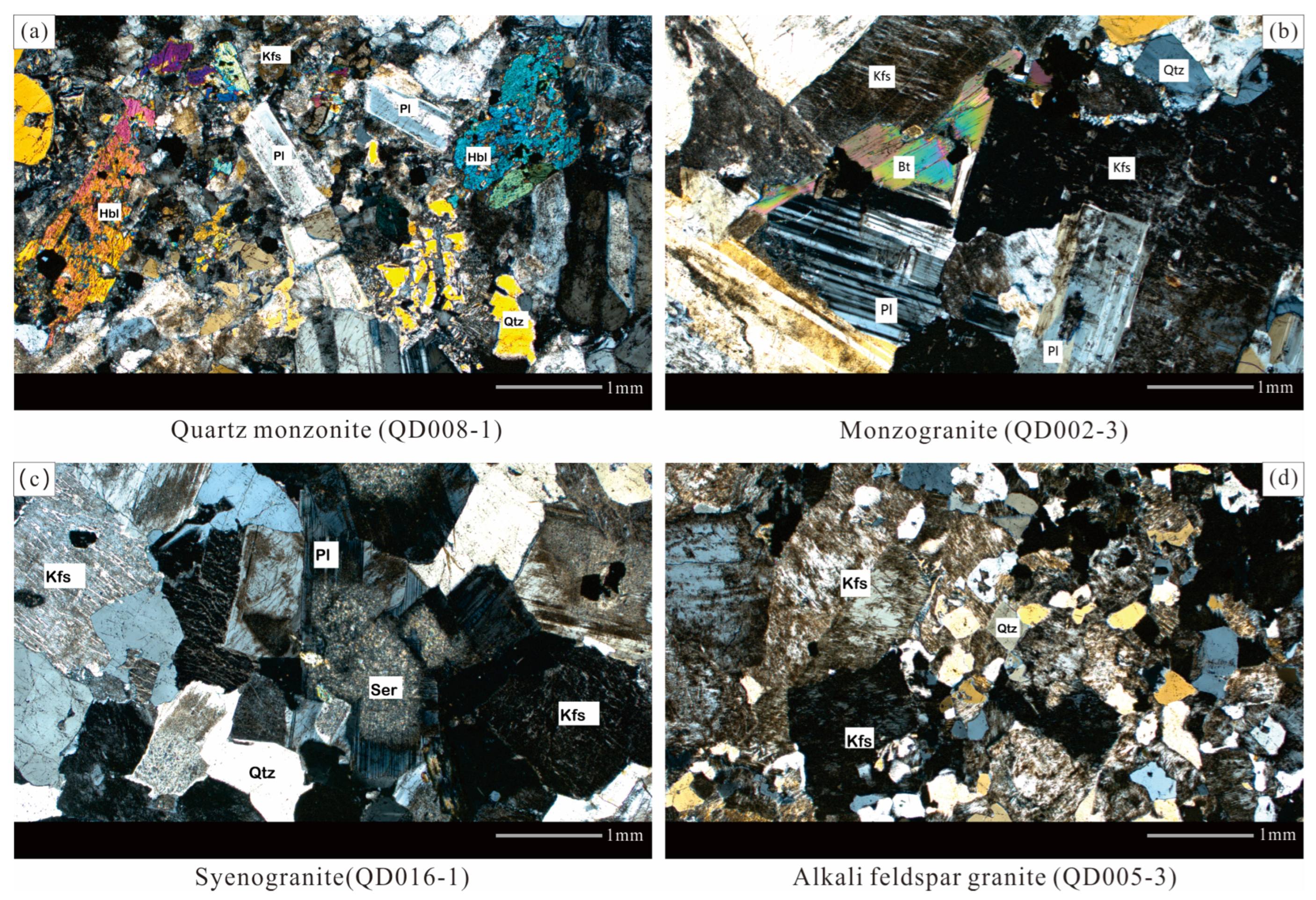The image features four small rectangular frames showcasing different types of minerals labeled from A to D. Each mineral is identified and unique in its coloration. 

- **Image A (Top Left):** This is Quartz Monzonite, labeled as QD008-1. It stands out as the most colorful, with hues of aqua, yellow, orange, hot pink, and purple.
  
- **Image B (Top Right):** This is Monzogranite, labeled as QD002-3. It features a less vibrant palette with blues, reds, bright purple, and yellows.
  
- **Image C (Bottom Left):** This is Cindergranite, labeled as QD016-1. It has a subdued mix of light blue, gray, black, and white.
  
- **Image D (Bottom Right):** This is Alkali Feldspar Granite, labeled as QD005-3, and is more colorful than Cindergranite with added yellows and blues, but still predominantly gray and white.

Each mineral displays a distinct range of colors and patterns, reflecting the diversity in their composition. The format of the images suggests a video presentation, adding a dynamic layer to the static nature of the minerals.